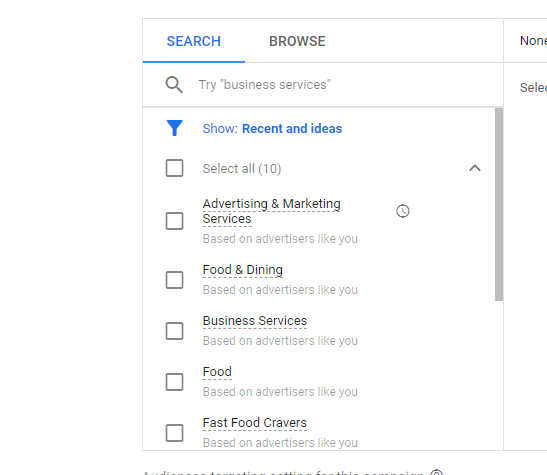The image captures an interface featuring a list with six checkboxes aligned on the left side. Next to the checkboxes are various search options and categories. The top left-hand corner of the interface includes a search bar with the text "Try business services" beside an icon of a magnifying glass. Below the search bar is an option labeled "Show recent ideas," indicating that the items listed are suggestions related to recent searches or interests. The list of categories includes "Food and Dining," "Business Services," "Food," "Fast Food," "Cravers," and "Advertising and Marketing Services." The overall background of the interface is white, while the text is in black, indicating a clean and user-friendly design likely intended for online or map-based service searches.